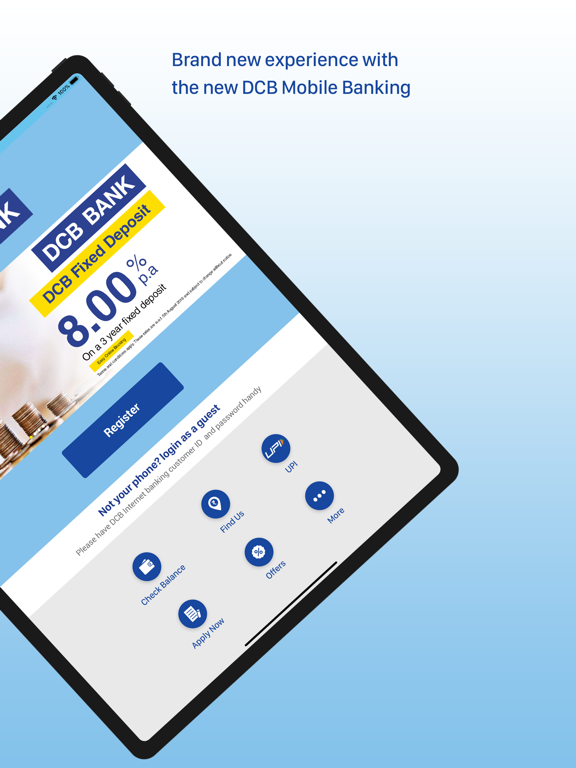A captivating visual showcases an ombre background transitioning from a very light sky blue at the top, almost white, to a darker yet distinct blue towards the bottom. In the middle of this gradient backdrop, bold dark blue text reads: "Brand New Experience with the New DCB Mobile Banking," with "NEW" and "DCB Mobile Banking" prominently capitalized.

An image of a tablet, possibly an iPad, is also featured but partially tilted, obscuring the upper left corner. Visible on the tablet's screen is the faint white letter 'K' at the top, followed by various information framed by navy blue and yellow rectangles. To the right of the 'K', a navy blue rectangle contains the white text "DCB Bank." Below it, a yellow rectangle displays the message "DCB Fixed Deposit" in blue text. The offer is highlighted with "8.00% P.A." in blue, and beneath it in black text, "Own a 3-Year Fixed Deposit."

Further down, a blue box with white text invites users to "Register." Subsequent options in blue text offer additional functionalities and information such as "Not Your Phone, Log In as a Guest," "Check Balance," "Find Us," "UPI Applied," and "Now Offers More."